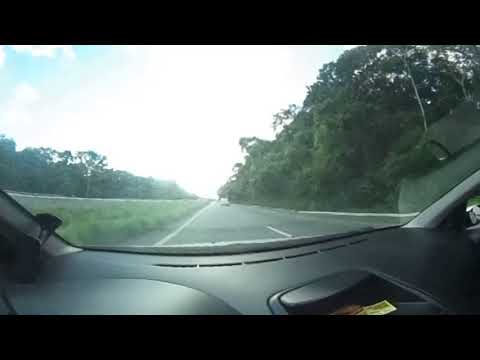This photograph, taken from inside a car, offers a clear view through the windshield and captures the perspective of someone seated on the left-hand side, likely the driver. The interior of the car features a black dashboard, with a small yellow and white tag visible on it. The scene outside portrays a divided highway with two lanes on each side, separated by a grassy median. The car is in the left lane of its two-lane road, following a white vehicle visible ahead. White dashed lines demarcate the lanes, guiding traffic flow. The road is flanked by tall green trees on either side, contributing to a rural interstate atmosphere. The sky presents a light blue hue in the top left corner, gradually transitioning to white on the right side, suggesting a bright, possibly sunny day with a hint of cloudiness in the distance.